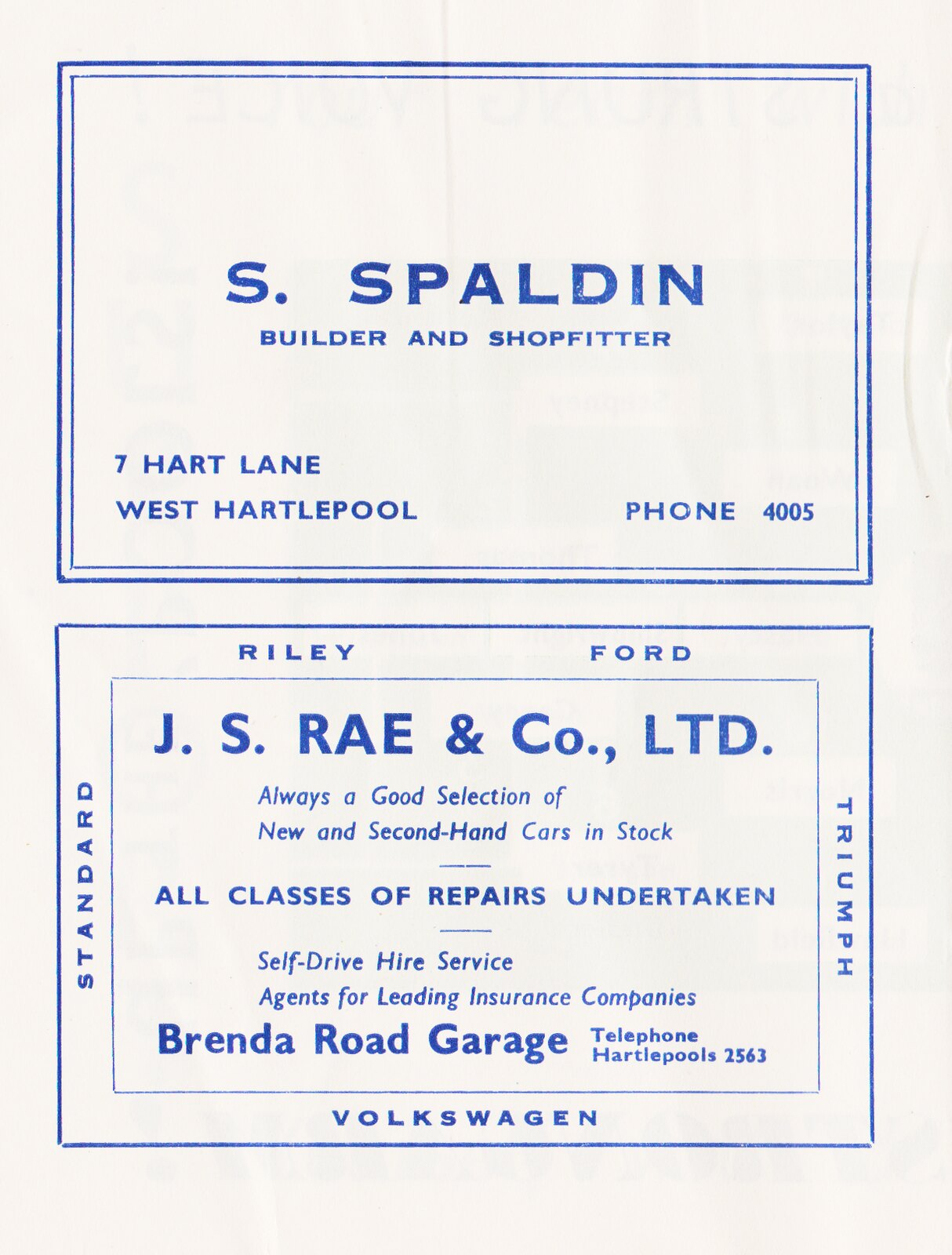The image features what appears to be a vertical magazine page showcasing two business advertisements. The ads are both bordered with thin blue frames against a white background and contain text in blue print. 

The top advertisement is for "S. Spalden, Builder and Shop Fitter." It is encased in a double blue border. Below the business name, the left corner provides the address: "7 Hart Lane, West Hartlepool," while the lower right corner displays the phone number: "4005."

The bottom advertisement has a single blue border and features several key elements:
- At the top of the ad, it's titled "Riley Ford."
- Prominently displayed in the center within a box is "J.S. Ray and Company Limited."
- Below that, smaller text reads: "Always a good selection of new and second-hand cars in stock."
- Further beneath, it states: "All Classes of Repairs Undertaken. Self-Drive Hire Service. Agents for Leading Insurance Companies."
- In larger print, it includes the contact information: "Brenda Road Garage Telephone Hartlepools 2563."
- The ad is flanked by the names of various car brands: "Riley Ford" at the top, "Standard" on the left, "Triumph" on the right, and "Volkswagen" at the bottom.

The style is typical of company ads, possibly resembling classified ads seen in newspapers or business flyers. The overall visual aesthetic is clear, functional, and text-heavy, aimed at providing detailed business information.